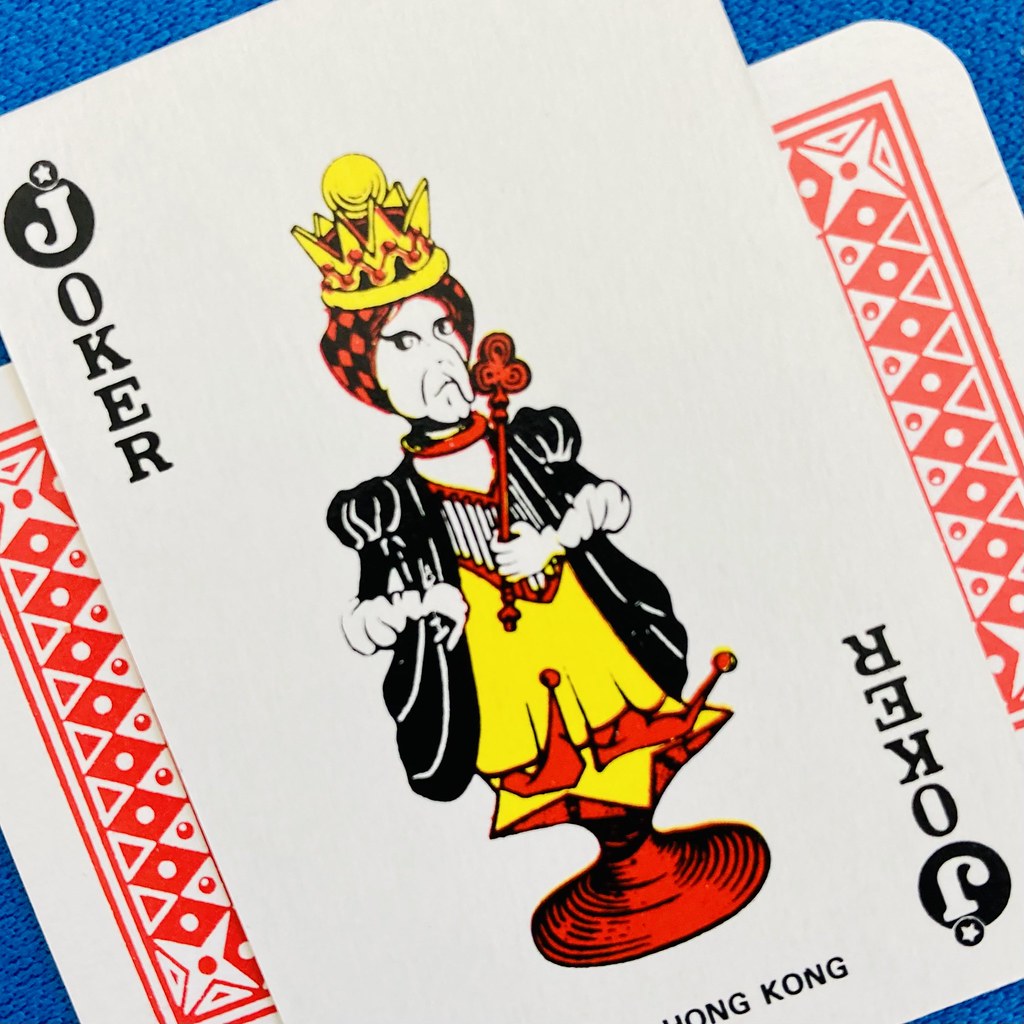Here's a refined and detailed caption for the image:

"This image displays a Joker card against a textured royal blue background, reminiscent of carpet or woven fabric, visible in all four corners. The card is placed at an angle, with one end directed towards the lower left corner and the other towards the upper right, though it doesn't reach the edge of the image. The card itself features a red diamond background accented by delicate white lines and white stars in the corners. Each red diamond has a white spot at the center, framed by a red border, and there are small red shapes, resembling squares or circles with a hint of white, interspersed between the diamonds. The top and bottom edges of the card are bordered by a continuous line.

The predominant focus of the card is the illustration of a Joker, portrayed as a queen with an exaggeratedly long nose and elaborate makeup, including elongated eyelashes and eyeshadow extending from the corners of her eyes. She dons a red and black kerchief and a notable yellow and red crown that rises in a zigzag pattern, each peak adorned with small balls, culminating in a larger yellow ball at the top.

In her left hand, she grasps a red scepter with three red circles at the top, reminiscent of the design of old skeleton keys. Her attire is a striking combination of a black jacket with puffy sleeves ending at the elbows, and a high-necked dress. The dress features a red collar, a white yoke with black stripes ending in a deep red V, and a yellow skirt extending to her feet. Her boots resemble those of a jester, ending in little balls.

She is positioned atop a red podium with rounded edges that flattens into a yellow star at the top. The bottom of the card includes the text 'Hong Kong', while 'Joker' is printed at both the top and bottom. The letter 'J' is enclosed in a black circle with a trademark symbol, consisting of a small white star inside another black circle above it, followed by the rest of the word 'Joker' in black letters."